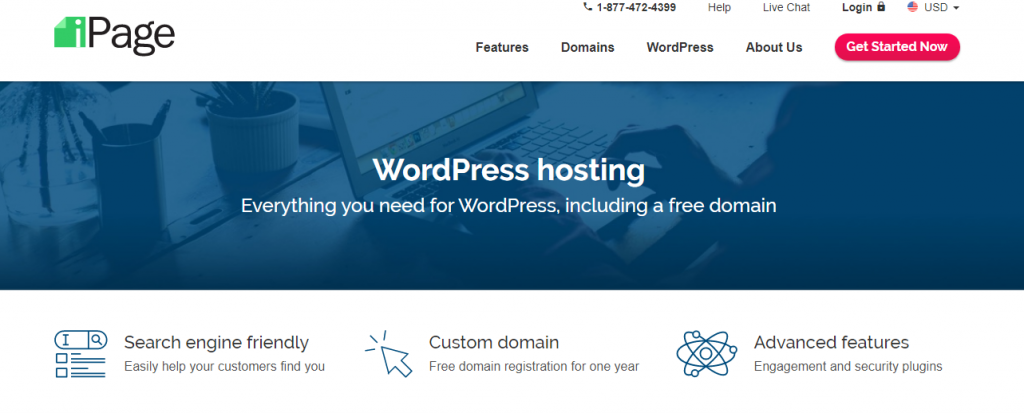Clipped Screenshot of a WordPress Hosting Service Web Page

The image is a clipped screenshot of a WordPress hosting service web page, showcasing a predominantly white background with blue accents and a notable blue banner in the center. Let's break it down from the top:

1. **Logo and Header**: At the very top is the iPage logo, featuring black text with a unique letter 'I' in white, overlaid on a folded green piece of paper. To the right of the logo, there is a phone number, options for help, live chat, login, and a currency switcher dropdown (defaulting to USD) accompanied by an American flag.

2. **Navigation Bar**: Below the header, there is a navigation bar with clickable pages including “Features,” “Domains,” “WordPress,” and “About Us.” To the right of these links is a prominent red button with white text that says "Get Started Now."

3. **Blue Banner Section**: Moving down to the center of the page, a blue banner displays a filtered image of a person typing on a laptop at a white desk. The desk also features a jar of pencils and a small pot with a plant. The overlay text on this banner reads: "WordPress Hosting - Everything you need for WordPress including a free domain."

4. **Icons and Options**: Beneath the blue banner, three cartoony icons illustrate key features of the service:
   - **Search Engine Friendly**: Represented by a mouse cursor over a search engine, indicating the platform's optimization for search engines.
   - **Custom Domain**: Symbolized by a clickable cursor, emphasizing the availability of custom domain options.
   - **Advanced Features**: Illustrated by a molecular structure drawing, suggesting the service offers advanced capabilities. Each icon is accompanied by brief explanatory texts consisting of four to six words. 

This detailed navigational and visual breakdown provides a comprehensive insight into the design and key offerings highlighted within this WordPress hosting service web page.